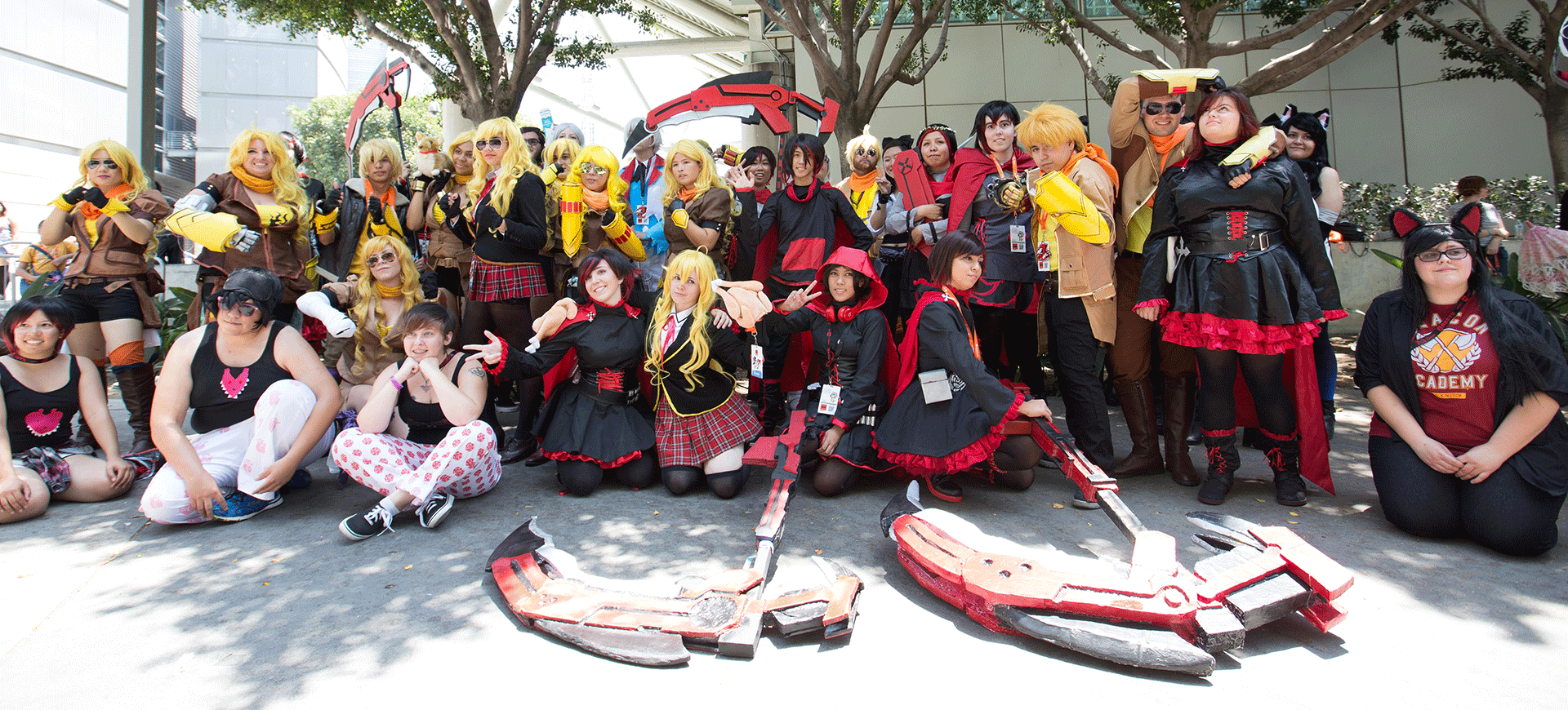This image captures a lively group of approximately 20 people, standing and seated on a sidewalk during a daytime costume convention, likely a Comic-Con. They are gathered underneath the shade of several green-leaved trees, which cast dappled shadows over the scene. The backdrop includes a white building with large glass windows, contributing to the urban setting.

The assembly features a diverse array of costumes, predominantly black with red accents. Many participants are cosplaying, with a noticeable presence of anime characters, including men dressed as women. Notably, there's an overweight woman on the far right, wearing a red shirt with "Academy" emblazoned on it, and black cat ears with red centers. She’s kneeling with her hands held in front of her stomach.

Central to the group are two individuals in black suits with red hoods, holding mechanical-looking weapons resembling axes with claws. Another distinctive figure is a man with white hair and a yellow sleeve. Towards the left, a cluster of participants with white hair in their costumes can be seen, along with three people in black tank tops. One person in this trio holds their chin up with a fist, while another reaches down towards a blue shoe. A young girl sits in the bottom left corner, with her hands placed behind her.

Many costumes feature frilly robe skirts and tank tops with pink emblems, evoking schoolgirl and magical girl aesthetics. Oversized costume weapons, including two large, custom red-and-black swords lying on the ground, add to the dramatic flair of the scene. Despite the variety of poses and outfits, there’s a clear sense of community and shared enthusiasm for cosplay in this vibrant gathering.